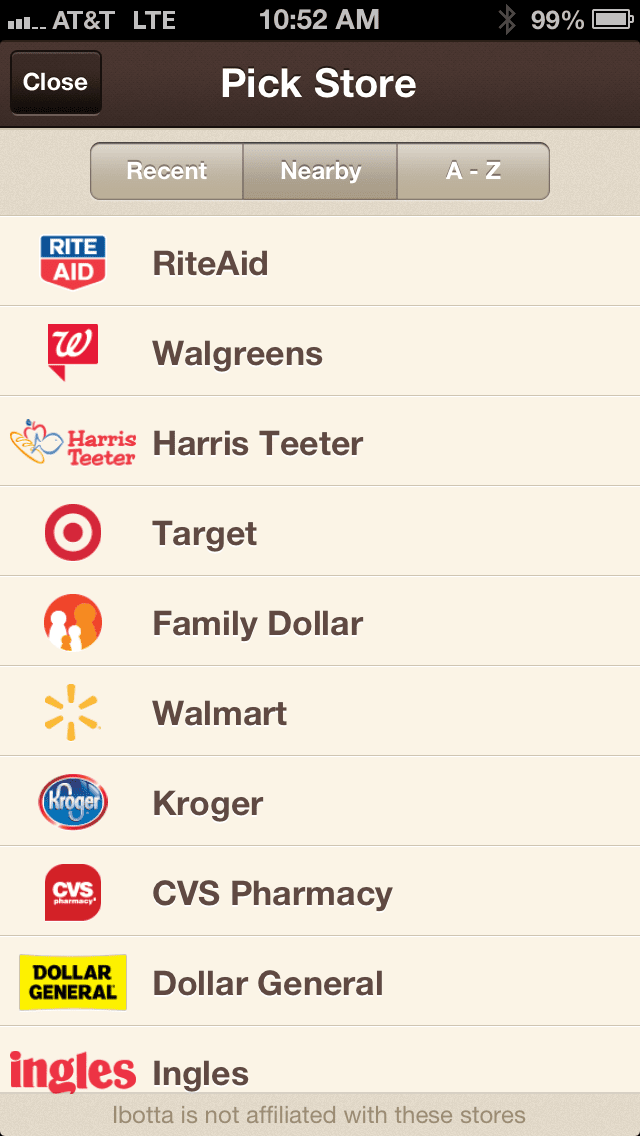The image depicts a screenshot of a cell phone displaying the Ibotta app interface. At the top-left corner of the screen, the status bar shows "AT&T," "LTE," the time "10:52 a.m.," and signal strength bars. On the top-right, it shows a battery icon with "99%" charge.

The app features a dark brown header with a white "Close" button on the upper-right corner, adjacent to the word "Close" also on a dark brown background. Below this header, the title "Pick Store" appears in white.

Three tabs labeled "Recent," "Nearby," and "A to Z" are displayed underneath in a lighter brown shade. The main part of the screen lists various stores, each separated by a line and named in brown text on a light brown background: "Rite Aid," "Walgreens," "Harris Teeter," "Target," "Family Dollar," "Walmart," "Kroger," "CVS Pharmacy," "Dollar General," and "Ingles." Each store name is accompanied by its respective logo, adding splashes of red, blue, yellow, and orange to the predominantly brown interface.

At the bottom of the screen, a disclaimer text in brown states, "Ibotta is not affiliated with these stores," indicating that the interface is part of the store-selection process for the Ibotta app.